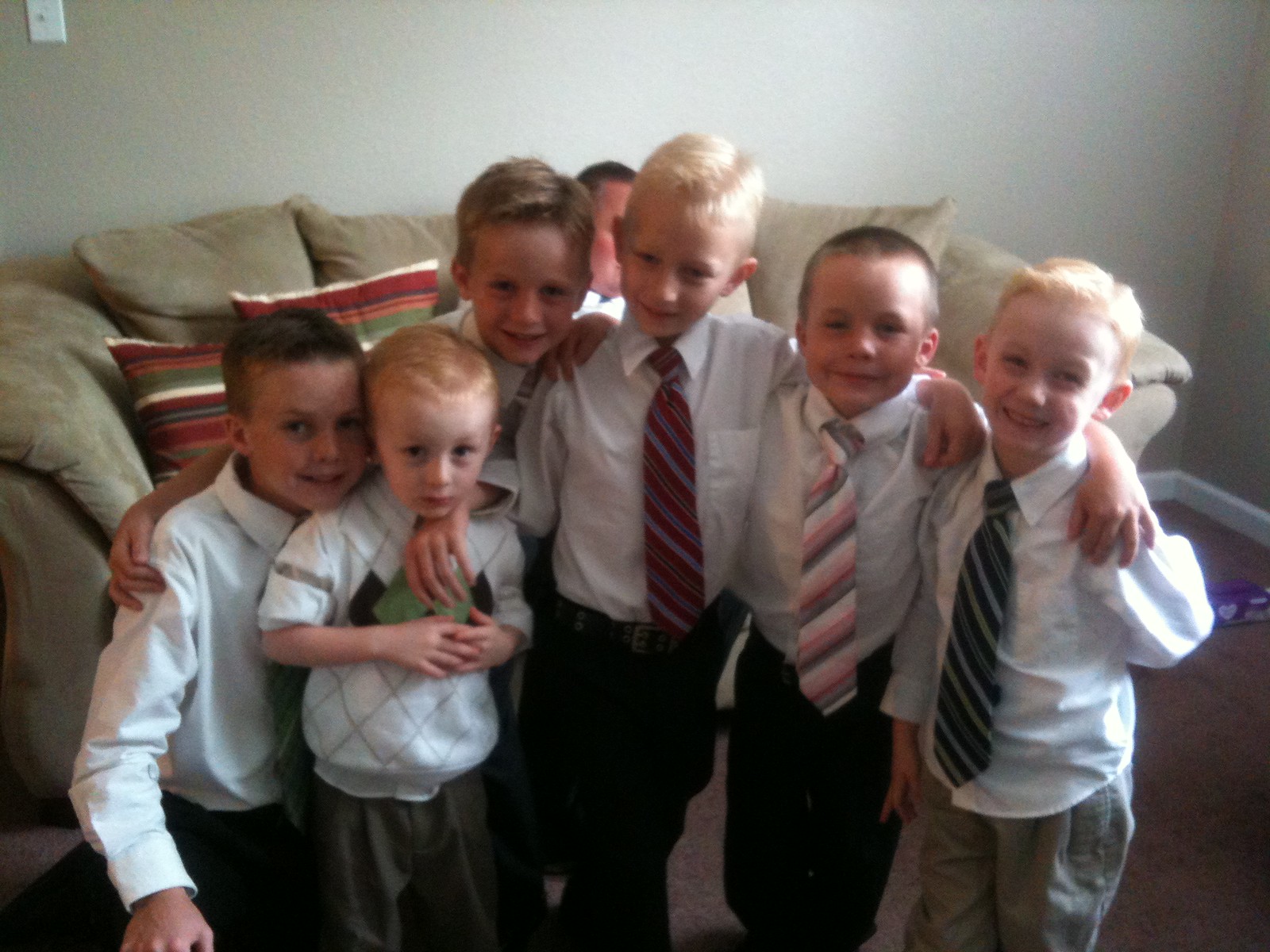In a cozy, well-lit living room with taupe-colored walls and an overstuffed beige couch adorned with two striped throw pillows, six young boys are gathered together, seemingly posing for a picture. The boys, all Caucasian and dressed in their Sunday best, range in age from about four to seven years old. Most of them wear long-sleeved white shirts with various colored striped neckties, while one of the younger boys, a redhead positioned in the front, sports an argyle short-sleeved sweater and chino pants. The background shows a glimpse of a chubby man with a red face and short-cropped hair sitting on the couch. The boys stand closely together, some with their arms around each other. The eldest, likely kneeling to fit into the frame, has brown hair, while the redheaded boy stands with his fingers intertwined in front. Behind them, a smiling boy with brown or blonde hair, a tall and slender toe-headed blonde boy with a red and gray striped tie, and a shorter boy with a buzz cut and a smirky grin wear ties of varying colors including gray, pink, white, green, and blue. The boys appear to be commemorating a special occasion, possibly right after a wedding reception or another formal event.